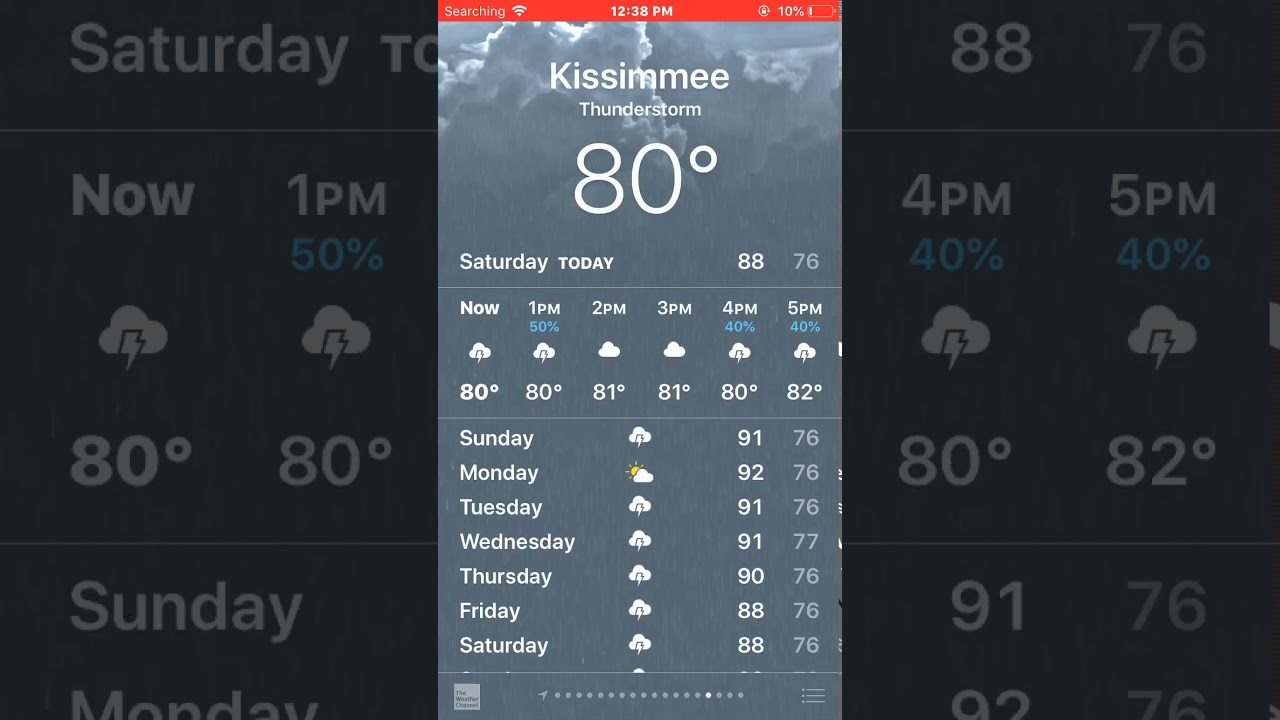The image is a computer screenshot featuring an embedded phone screenshot at its center. The overall background of the image is dark and displays an enlarged version of an hourly weather forecast. This background highlights the current time slots from "Now" through "4 PM," corresponding to the weather updates provided.

At the focal point, the phone screenshot prominently shows several alerts and pieces of information: 
- A red bar at the top indicates "Searching for signal."
- The current time is displayed as "12:38 PM."
- The phone battery icon reveals a critical 10% remaining charge.

Beneath these notifications, the weather details are specific to "Kissimmee." The temperature at the moment is 80°F with a thunderstorm, illustrated by icons and descriptive text. The day's forecast includes:
- "Saturday Today: High of 88°F, Low of 76°F."
- Hourly updates detail:
  - "Now: 80°F with lightning, 50% chance of thunderstorms at 1 PM."
  - "1 PM: 80°F, 50% chance of lightning."
  - "2 PM: 81°F."
  - "3 PM: 81°F."
  - "4 PM: 40% chance of thunderstorms, 85°F."
  - "5 PM: 40% chance of thunderstorms, 82°F."

Looking ahead, the forecast lists daily high and low temperatures for the next week:
- "Sunday: High 91°F, Low 76°F"
- "Monday: High 92°F, Low 76°F"
- "Tuesday: High 91°F, Low 76°F"
- "Wednesday: High 91°F, Low 77°F"
- "Thursday: High 90°F, Low 76°F"
- "Friday: High 88°F, Low 76°F"
- "Saturday: High 88°F, Low 76°F"

The repeated background denotes the current and upcoming hourly forecasts from "Now" through "4 PM," amplifying the same segments detailed within the central phone display, thus creating a layered, detailed look at the weather information.